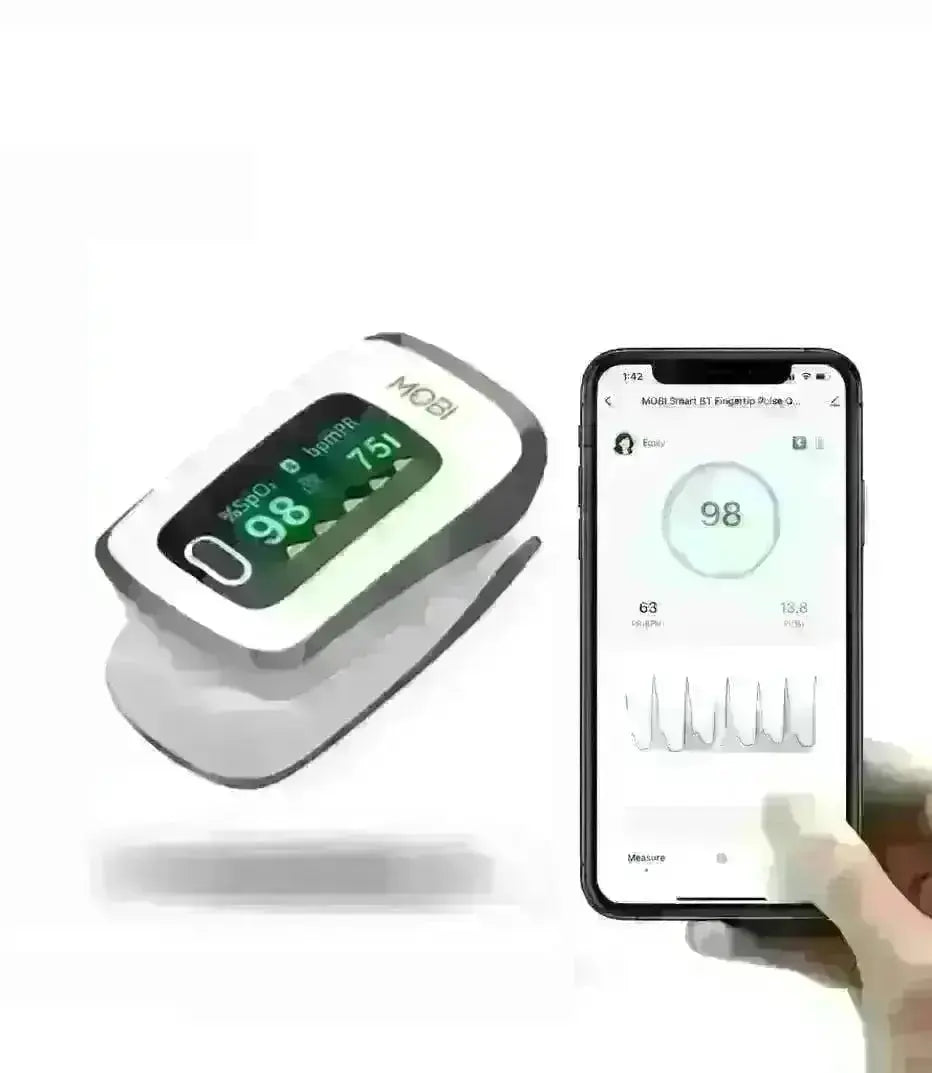The image features a detailed view of two devices: a small, rectangular blood pressure monitor on the left and a smartphone on the right, held by a hand. The monitor, with its primarily white body outlined in black, displays readings in bright green text on a black screen. Key information includes "%SPO2 98" and "BPMPR 75," with the top of the screen displaying "M-O-B-I" in black capital letters. The smartphone screen shows a detailed interface labeled "Mobile Start BP Fingertip," featuring a circle with "98" inside, smaller readings of "63" to the left and "13.8" to the right, and a heart monitor line at the bottom. The predominant colors in the image are white, black, and shades of green, and while the image is somewhat blurry, the primary elements and text remain clear.